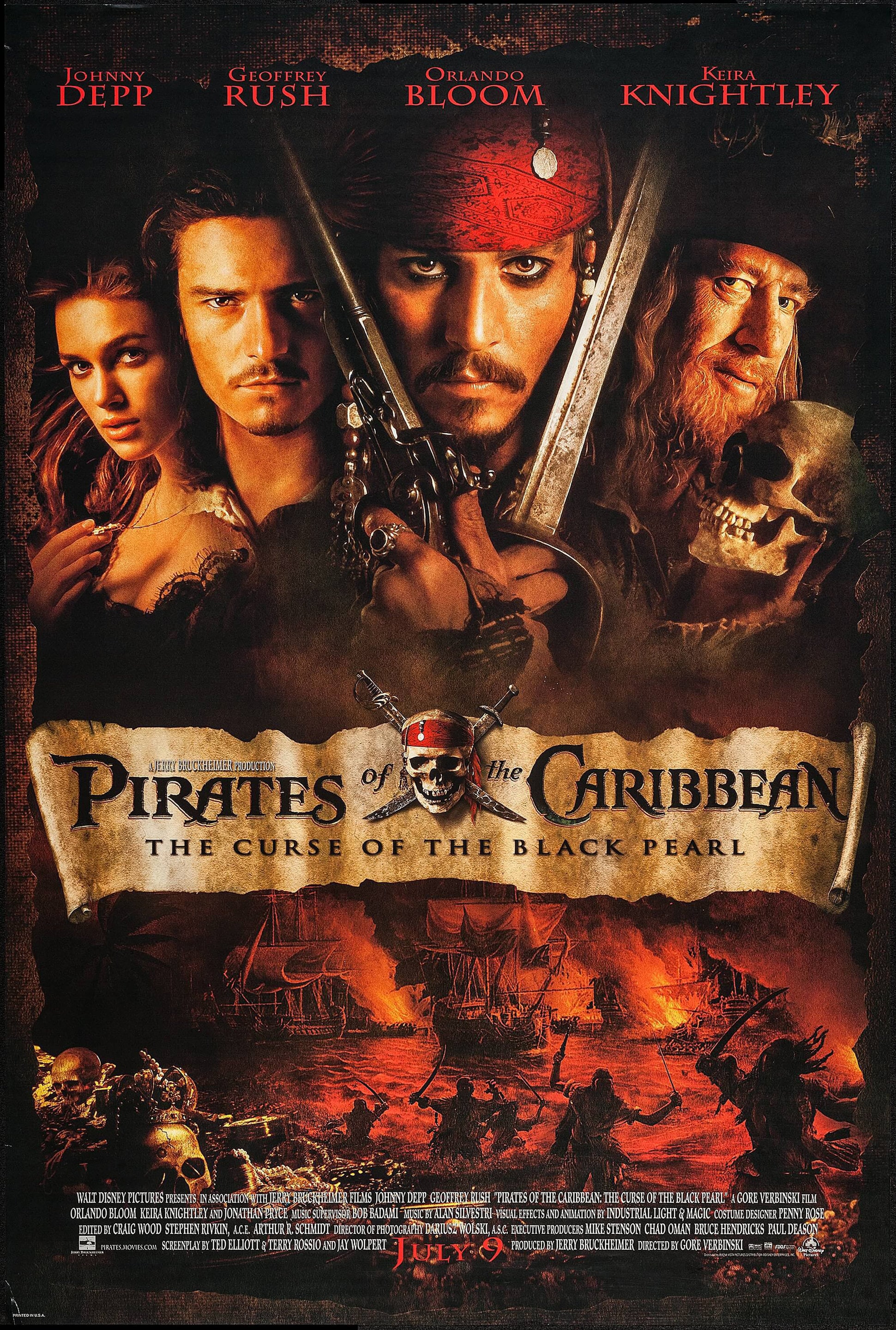This is a detailed movie poster for "Pirates of the Caribbean: The Curse of the Black Pearl." The background of the poster is predominantly dark, creating a dramatic effect. Centered at the top of the poster, the names of the main cast—Johnny Depp, Geoffrey Rush, Orlando Bloom, and Keira Knightley—are written in red letters. Their portraits are arranged below this text, with Johnny Depp as Captain Jack Sparrow prominently in the center, holding a sword and a gun, and wearing a red head wrap. Flanking him are Orlando Bloom and Geoffrey Rush, with Keira Knightley's portrait to the far left.

Beneath these portraits, the title "Pirates of the Caribbean: The Curse of the Black Pearl" is displayed on a weathered scroll, featuring a skull and crossbones emblem. The lower portion of the poster illustrates a dramatic and chaotic scene of pirate ships engulfed in flames, with silhouettes of men emerging from the water brandishing swords, symbolizing intense pirate battles. To the left, there is an antique treasure chest overflowing with gold and skulls. Additional details such as the director's name and other credits are written in white at the bottom.